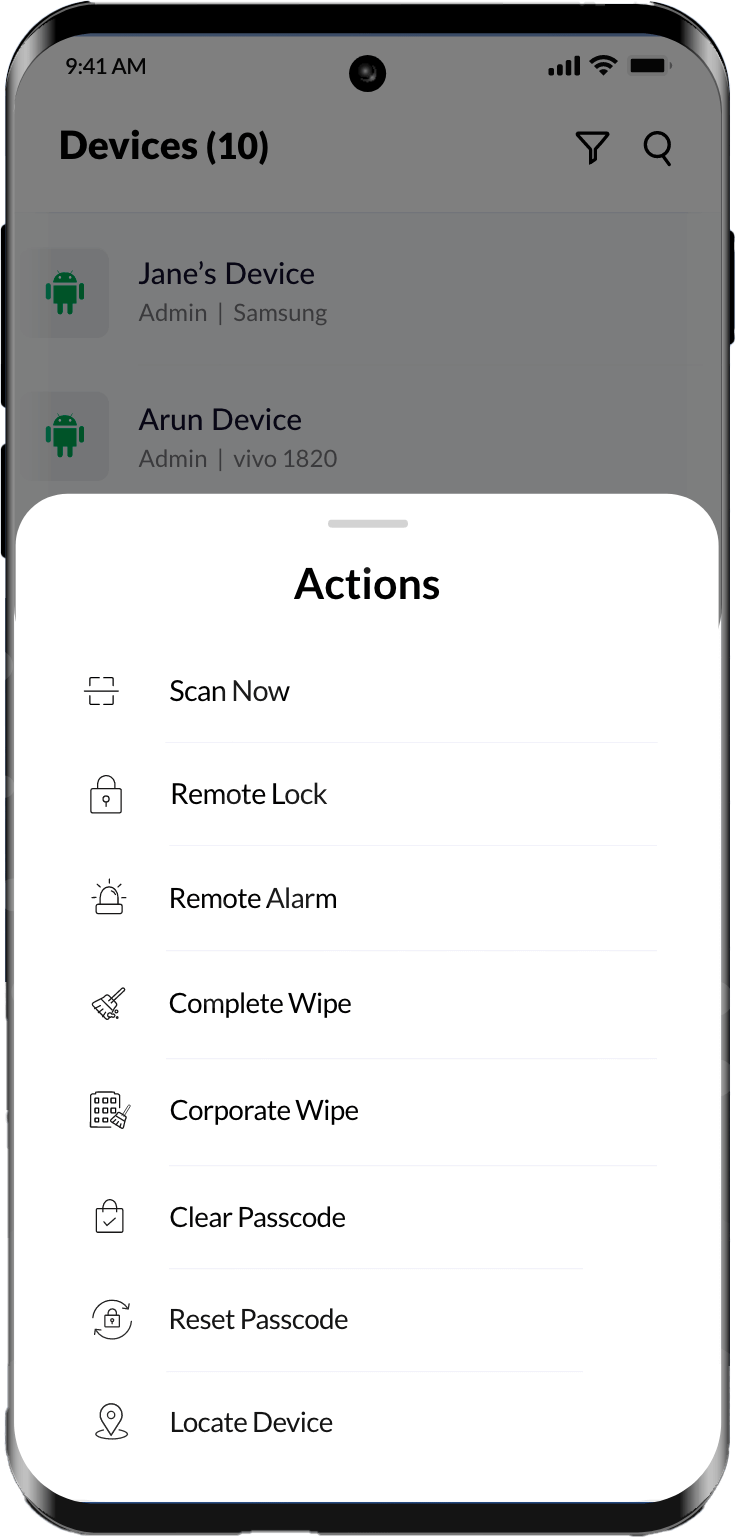The image appears to be a mock-up of an Android smartphone, showcasing a screenshot within the device's bezel. The phone features external buttons typical of Android devices and includes a front-facing camera, four signal bars, full Wi-Fi connectivity, and a fully charged battery, with the timestamp showing 9:41 AM.

The screenshot itself depicts a corporate application designed to manage and monitor company-owned Android devices. The main menu lists various devices, including "Jane's Device" and "Aaron's Device," with corresponding admin labels such as "Samsung" and "Vivo 1820." The interface allows for multiple actions: "Scan Now," "Remote Lock," "Remote Arm," "Complete Wipe," "Corporate Wipe," "Clear Passcode," "Reset Passcode," and "Locate Device."

At the top of the screen, there is a search bar and filter menu, indicating potential functionalities for sorting and finding specific devices within the fleet. However, the mock-up reveals some editing imperfections, particularly where the screenshot is integrated into the phone's bezel. The edges are poorly cropped and appear jagged, lacking proper anti-aliasing, which detracts from the realism of the mock-up.